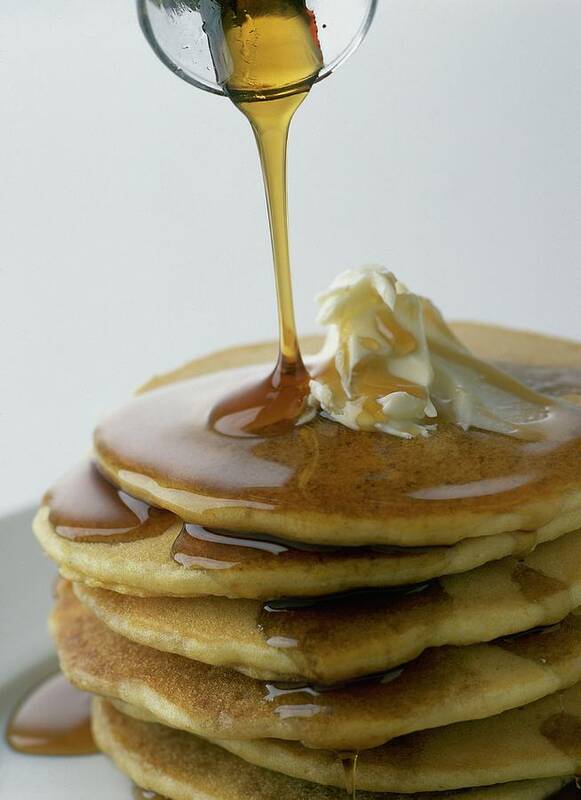In this detailed close-up photograph, a delectable stack of six golden-brown pancakes is showcased, each layer appearing fluffy and well-cooked. Atop the stack, there's a generous mound of creamy, melting butter. The photograph captures the moment syrup, amber in color, is being poured from a clear glass bottle, which is only partially visible at the top edge of the image. The syrup cascades down the sides of the pancakes, creating a glistening trail that drips onto the white plate below, where a small puddle has formed. The background is a clean, almost indistinguishable out-of-focus white, drawing full attention to the mouthwatering breakfast treat. The overall composition and sharpness of the image give it a polished, appetizing appeal, akin to a restaurant advertisement.